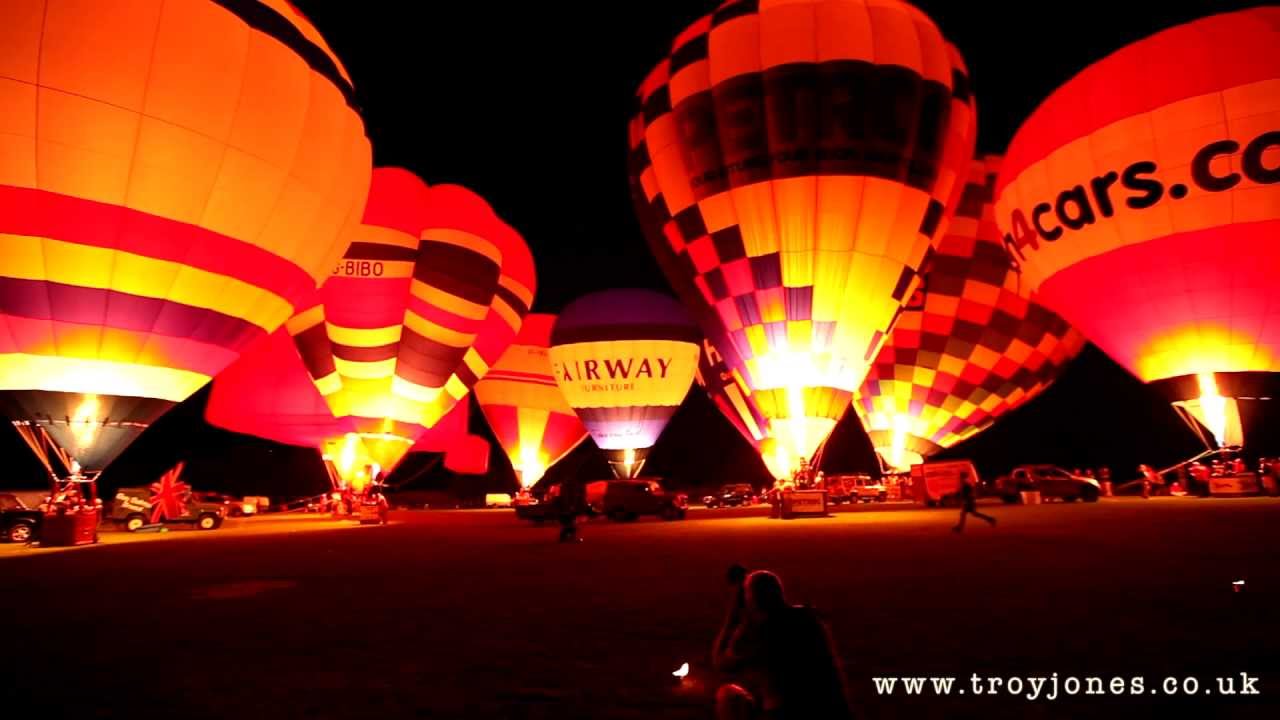The image captures a nighttime scene of multiple hot air balloons in the process of being inflated. The sky is pitch black, and the only light source comes from the flames underneath the balloons, casting a golden, reddish hue over the scene. The balloons themselves are large and still tethered to the ground, with their baskets awaiting lift-off. Several feature striking designs, including checkered patterns, adding to the visual interest. Some balloons display website names like airway or acars.com. In the bottom right corner of the image, there is a small overlay with the text "www.troyjones.co.uk," identifying the photographer.